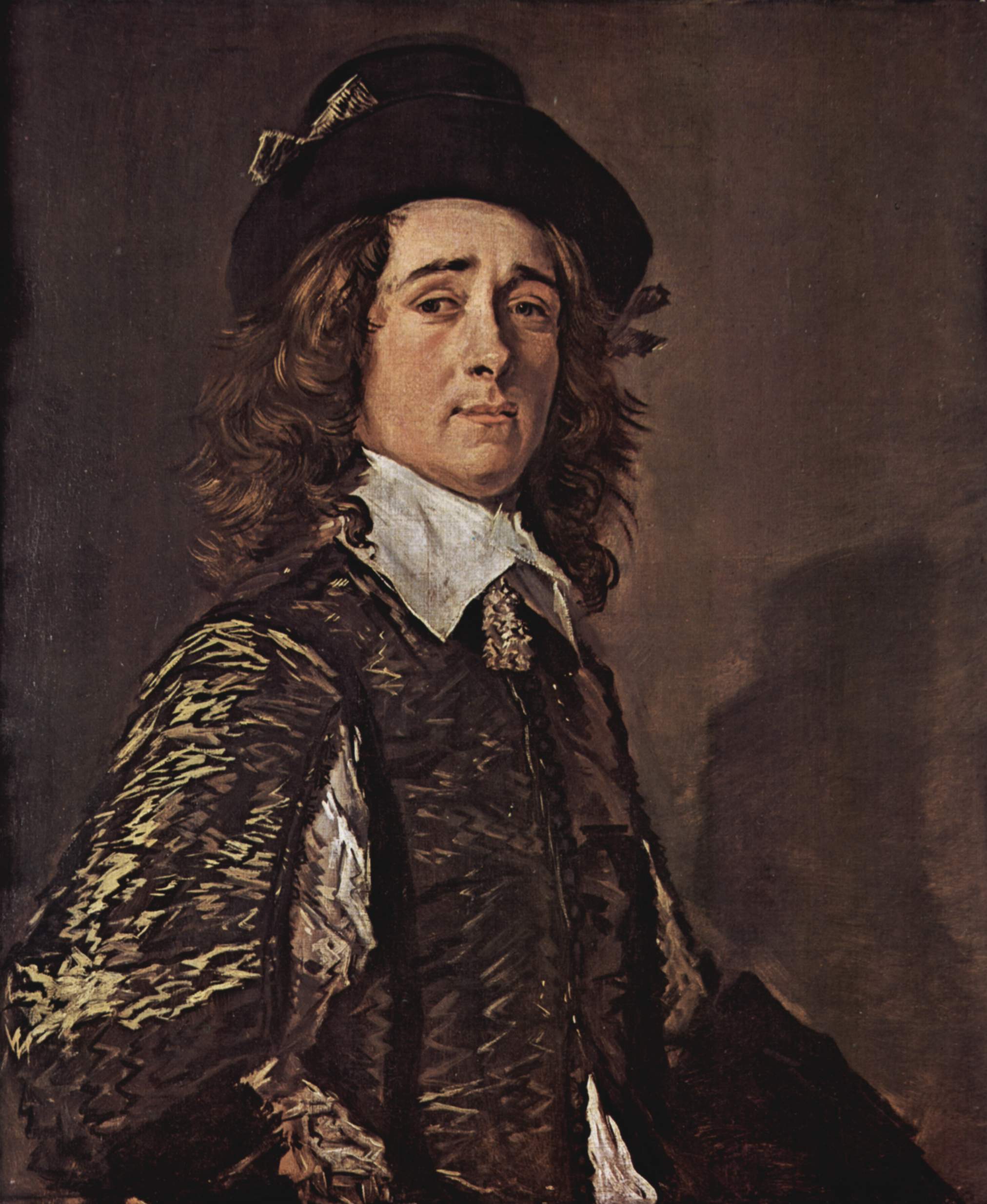This Renaissance-style painting portrays a wealthy and distinguished man with long, wavy brown hair cascading below his shoulders. He wears an elegant black hat adorned with a gold bow, adding to his sophisticated allure. His hair compliments his serious yet dignified expression, emphasized by his piercing eyes gazing down to the left. His white, ruffled collar prominently features a gold ornament hanging below, while his attire consists of an elaborate and richly designed dress shirt with patterns of gold, white, and black, akin to a suit coat from a bygone era. The painting, a vertical rectangle, captures the man from his waist up, showing him sitting upright with his chest turned to the right. Despite this, his face looks forward into the onlooker’s gaze, surrounded by a background of a muted brown wall with a stark black shadow cast behind him, accentuating his presence.